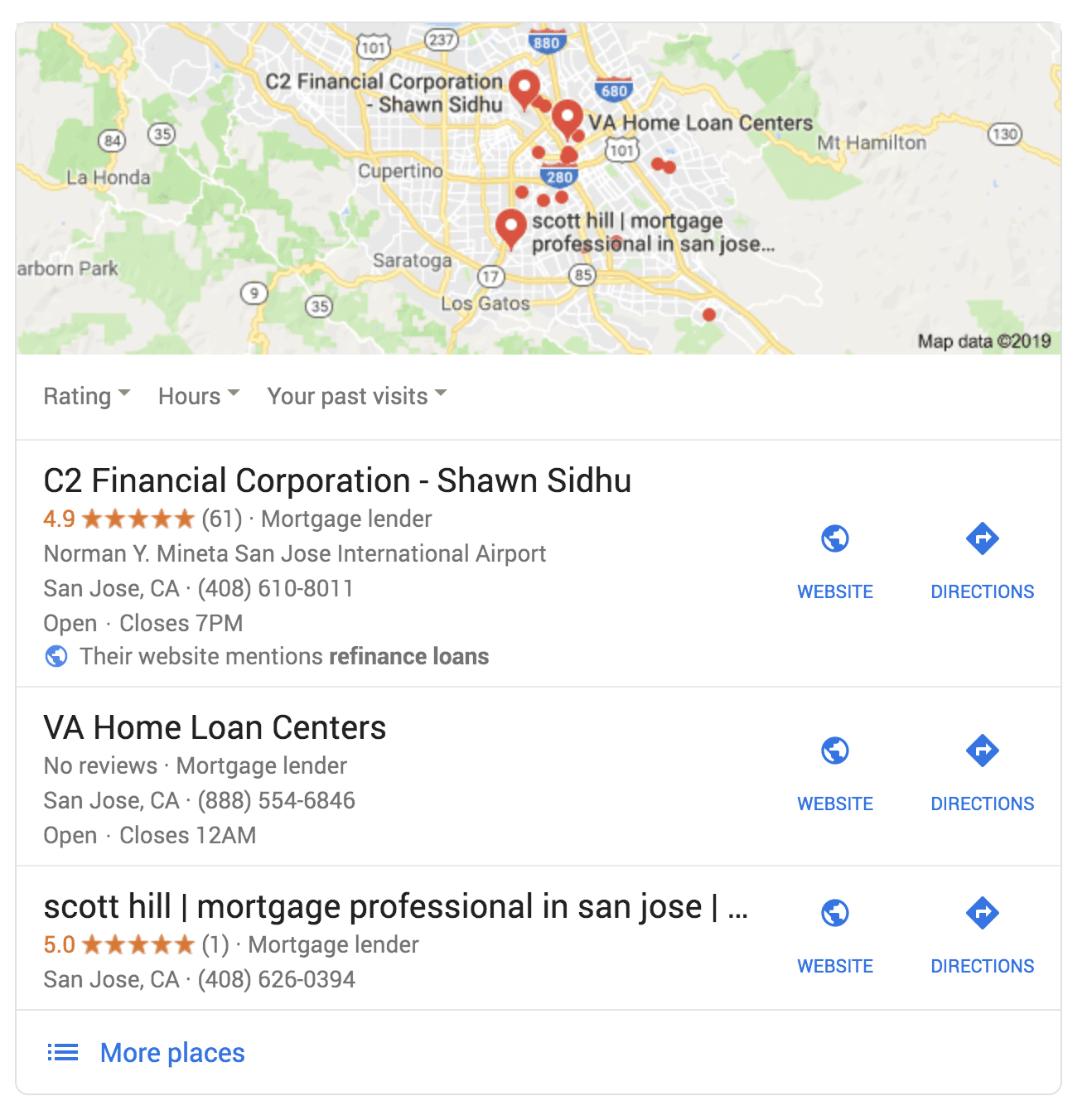This image displays the search results for financial and loan centers in San Jose, California. At the top of the results page, a map is prominently featured with several red pins indicating the locations of the relevant businesses. Below the map, three businesses are listed: 

1. **C2 Financial Corporation, Sean Sidhu**
2. **VA Home Loan Centers**
3. **Scott Hill Mortgage Professional, San Jose** 

These businesses appear to specialize in home loans and mortgages, offering various financial services such as lending, mortgages, and refinancing. Each listing includes a button to visit the business's website and another button for directions to the physical location of the business. This setup allows users to either explore the services online or visit the centers in person for further assistance.